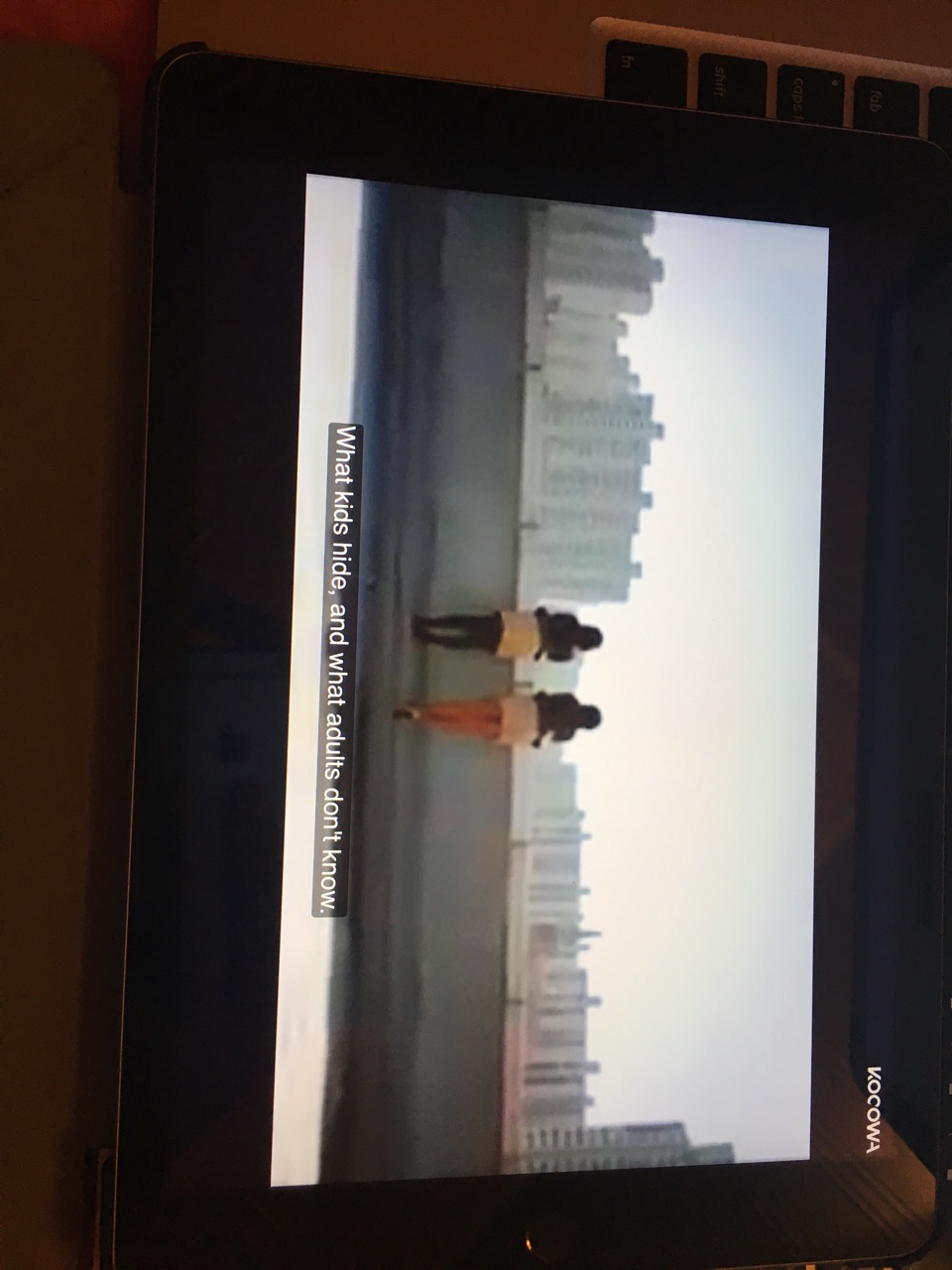The image captures a scene that could almost be straight out of a movie, with a distinctive feel that makes it hard to tell whether it's a photo or a stylized drawing on a screen. Framed in black, the picture is turned on its side and viewed through a smartphone. It shows two figures, possibly a parent and child, standing side by side on a rooftop or a bridge with a waist-high railing, facing away from the camera. Both wear identical hoodies—black on the top and beige on the bottom. One person is dressed in black leggings and black shoes, while the other wears a dress with salmon-colored leggings and white shoes. They overlook a cityscape of skyscrapers and large buildings under an overcast sky. Subtitles at the bottom of the image read, "what kids hide and what adults don't know." This adds a poignant narrative layer to the otherwise tranquil but contemplative scene.